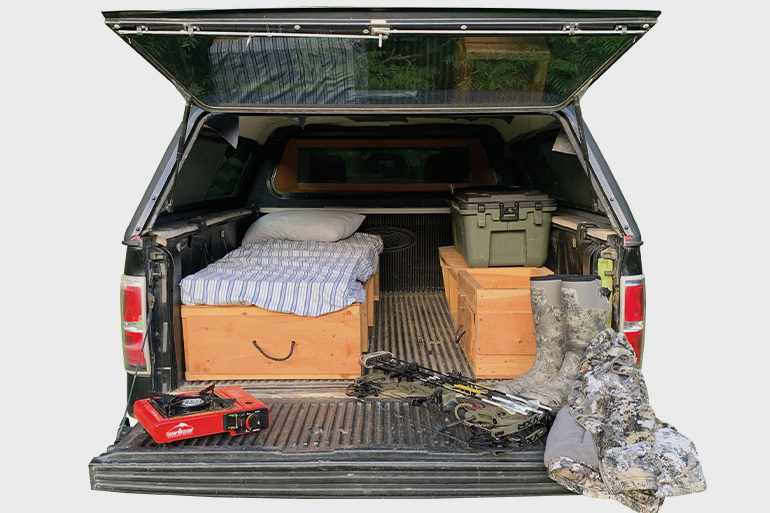This photograph captures the back of a covered, dark gray truck bed, where an outdoor living setup is evident. The truck's tailgate is open, revealing a cozy makeshift camping arrangement inside. A small, bed-sized mattress, adorned with blue and white striped sheets and a white pillow, is placed atop medium beige wooden boxes, creating a raised sleeping area that appears slightly smaller than a typical twin bed. To the right of the bed, a wooden trunk supports an army green cooler, contributing to the organized storage solution. Scattered across the tailgate and inside the truck bed are various hunting and camping essentials: camo boots, a camo coat, arrows for a bow, and a red propane cooker. This practical and rustic setup suggests the truck belongs to someone who uses it as a base for hunting or outdoor expeditions. The worn look of the items and the truck give the impression of a well-used and cherished mobile campsite.